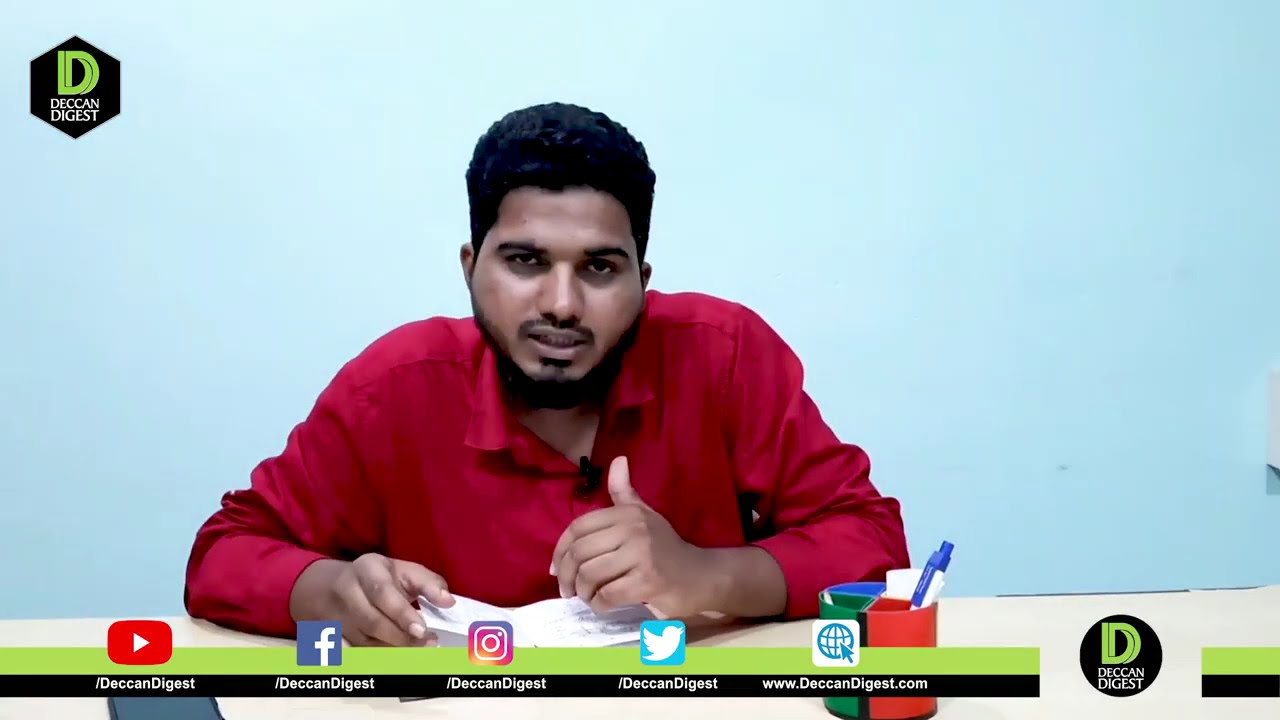In this image, a man of likely Middle Eastern or South Asian descent with darker skin, black hair, a well-trimmed black beard, and a thin mustache is seated at a white desk. He appears professional, wearing a red button-up shirt with a microphone attached at the bottom of the V-neck. The man is holding a piece of paper in one hand, with his other hand placed on top of it, and he is looking forward as if he is speaking. In front of him, there is a cup holder containing various markers. The background of the image is a baby blue tone.

In the top left corner, there is a black hexagon logo containing a bright green letter "D" and the text "Deccan Digest" written in white letters. The same logo appears in a circular form in the lower right corner of the image. Spanning across the bottom of the image is a banner displaying social media icons and the handles for Deccan Digest on YouTube, Facebook, Instagram, Twitter, along with the website link www.decondigest.com. The man’s focused expression and the setup suggest he is part of a professional recording or broadcast for Deccan Digest.